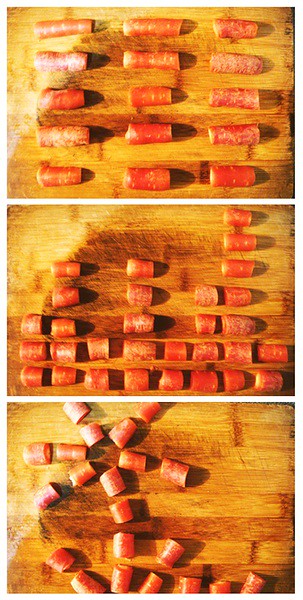The image displays a series of three photographs stacked vertically, each showcasing an array of chopped pieces of what appears to be Chinese sausage or possibly old, dried carrots, all presented on a yellow-brown wooden cutting board. In the top image, there are exactly 15 pieces arranged neatly in a grid of three rows and five columns. The middle photograph features around 30 smaller pieces, lined up with less uniformity, creating a slightly irregular pattern. The bottom image showcases these small pieces arranged in a spiral formation, intertwined closely together. Each section of the montage has a distinct yet harmonious orange hue, highlighting the meticulous arrangement and the textured surface of the cutting board beneath.